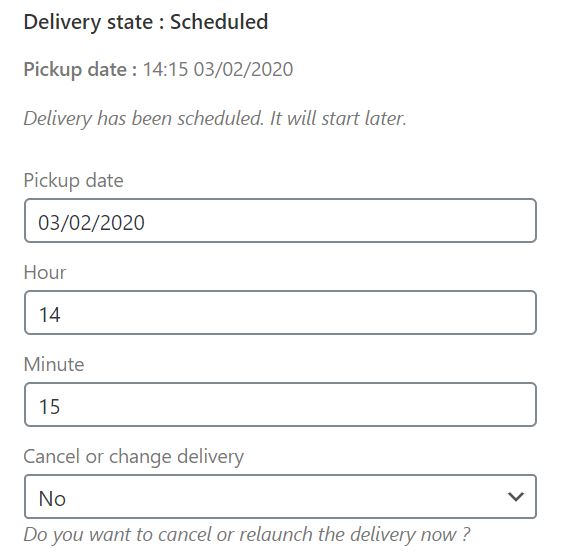A detailed caption for the described image could be:

"This image, likely captured from a computer or cell phone screen, displays a user interface related to delivery scheduling. At the top of the screen, it reads 'Delivery State: Scheduled.' Below this, starting from the left and moving right, the text 'Pickup Date: 14:15 03/02/2020' is visible. Further down, there is a notice stating, 'Delivery has been scheduled and will start later.' 

Additionally, there is another section with the label 'Pickup Date: 03/02/2020,' with corresponding time fields indicating 'Hour: 14' and 'Minute: 15.' Next to this, there is an option labeled 'Change or Cancel Delivery,' followed by a drop-down arrow indicating that the user can alter this selection. The current setting is 'No,' but the drop-down implies it can be changed to 'Yes.'

Beneath this, a prompt asks, 'Do you want to cancel or relaunch the delivery now?' with a question mark at the end. 

The interface features long, skinny bars or rectangles, many of which are only partially filled by the text responses, leaving significant empty space."